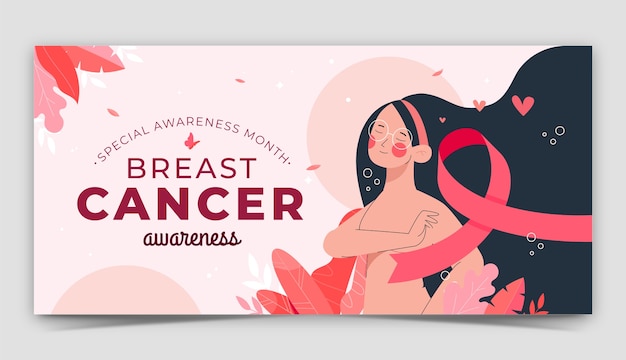The image is a slightly wider-than-normal business card or flyer set against a grey background, featuring a cohesive color palette of varying shades of pink, pinkish-orange, and mauve. On the left side of the card, in a semi-circle layout, the text "Special Awareness Month" is prominently displayed. Below this, the phrase "Breast Cancer Awareness" is written, accompanied by an illustrated butterfly. In the top left-hand corner, there are three multicolored leaves. Scattered throughout the design are additional elements such as leaves, hearts, and bubbles, contributing to the card's delicate and whimsical aesthetic.

On the right-hand side of the card, there is a cartoon illustration of a woman with black hair, wearing glasses and a pinkish-red headband. A breast cancer awareness ribbon partially stretches across her body and hair. The woman, depicted without visible clothing, has her right arm folded across her chest, modestly covering her breasts. She is surrounded by more leaves at the bottom of her figure and has her eyes closed with a gentle smile on her face. Delicate hearts and bubbles are illustrated around her hair, enhancing the card's overall charm and thematic unity.